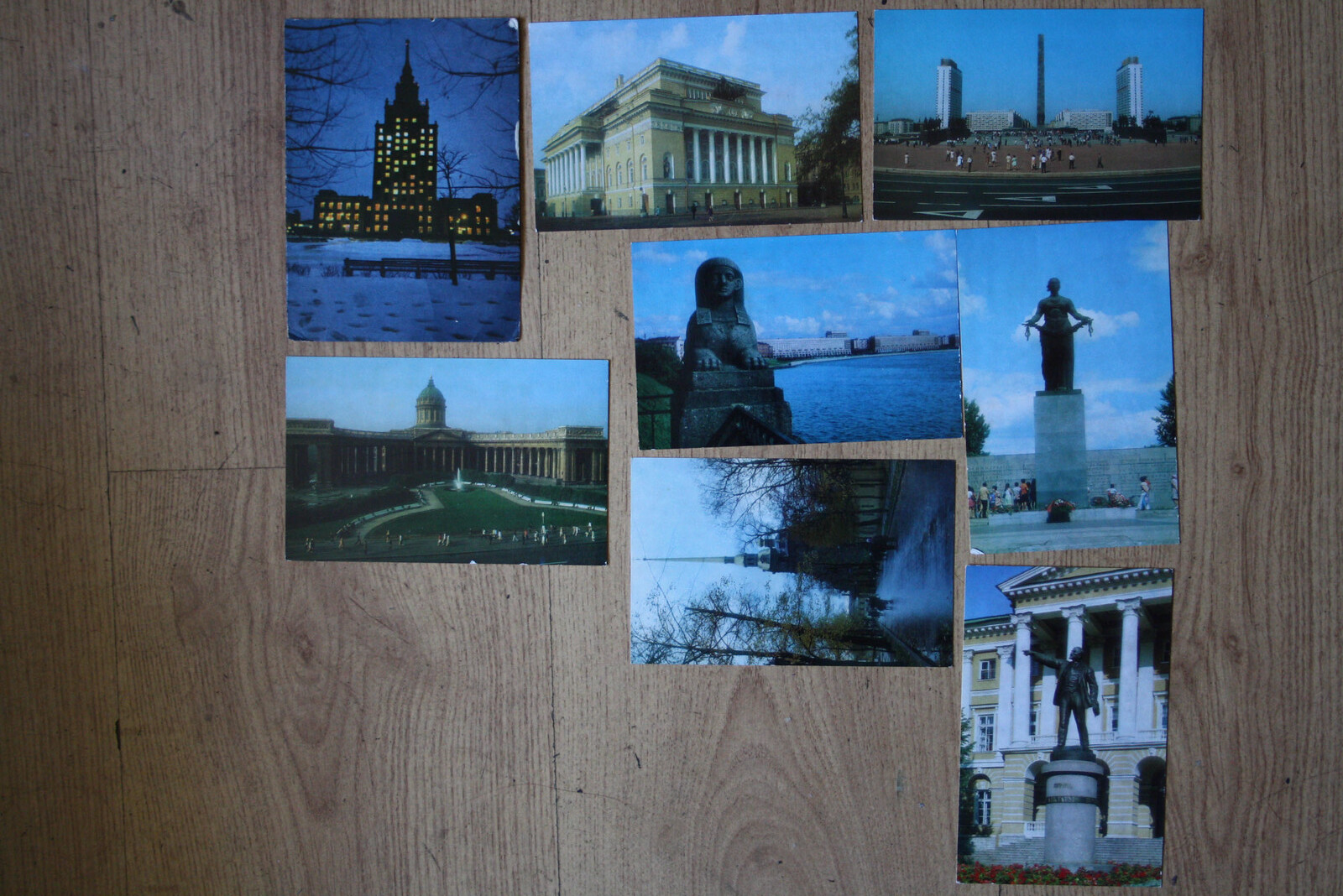The image features a collection of photographs displayed against a light brown paneled wall, characterized by large, vertical wooden panels. The photographs, resembling postcards, showcase various monuments and notable buildings from around the world, arranged on a horizontal line. Starting from the left, there is a noticeable gap before the photos begin. 

The top-left photograph is vertically oriented, showcasing a city building illuminated by snow and surrounded by yellow lights. To the right of this building is an iconic Pantheon structure, oriented horizontally. Below it, there are images of various cityscapes, including a courtyard with statues positioned vertically.

In the center of the arrangement is a striking photograph of a sphinx-like stone statue near an island or pond. To the right of this central image is another monument topped with a statue. Further to the right, a prominent vertical photograph depicts several skyscrapers.

At the bottom-left, there is a horizontally oriented photograph of a significant government building with a large courtyard, though it is turned 90 degrees to the left. Moving rightwards, additional photographs depict statues, including one at the bottom right-hand side, which features a statue in front of a white building.

Overall, this indoor photograph captures a curated array of global architectural marvels and statues, set against a warm, wooden backdrop without any text to identify the subjects precisely.